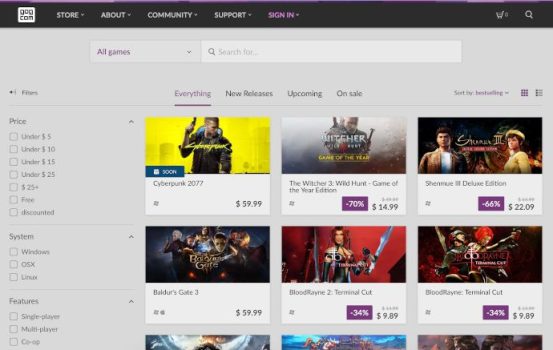This screenshot from GOG.com, an established online game store known for offering a variety of digital game purchases, provides a detailed view of the website's interface and highlighted offerings. The top navigation bar includes links to "Store," "About," "Community," "Support," and a "Sign-In" option, which is highlighted in purple. Accompanying these are icons for searching the site and accessing the shopping cart situated in the top right corner.

Directly below the navigation menu, a drop-down menu labeled "All Games" allows users to filter game listings by categories. The left sidebar features numerous filter options, such as price ranges ("Under $5," "Under $10," "Under $15," "Under $25"), system compatibility (Windows, OSX, Linux), and game modes (Single Player, Multiplayer, Co-op).

Displayed prominently in the game listings are several notable titles: 
- "Cyberpunk 2077" priced at $60
- "The Witcher 3" at a 70% discount, available for $14.99
- "Shenmue III Deluxe Edition," 66% off at $22.09
- "Baldur's Gate 3" priced at $60
- "BloodRayne 2: Terminal Cut," 34% off at $9.89
- "BloodRayne: Terminal Cut," similarly discounted at 34% for $9.89

The bottom section of the screenshot includes partial images of three additional game listings, whose details are obscured. This comprehensive display underlines GOG.com's diverse portfolio and user-friendly interface, reinforcing its reputation as a legitimate and versatile platform for purchasing games.